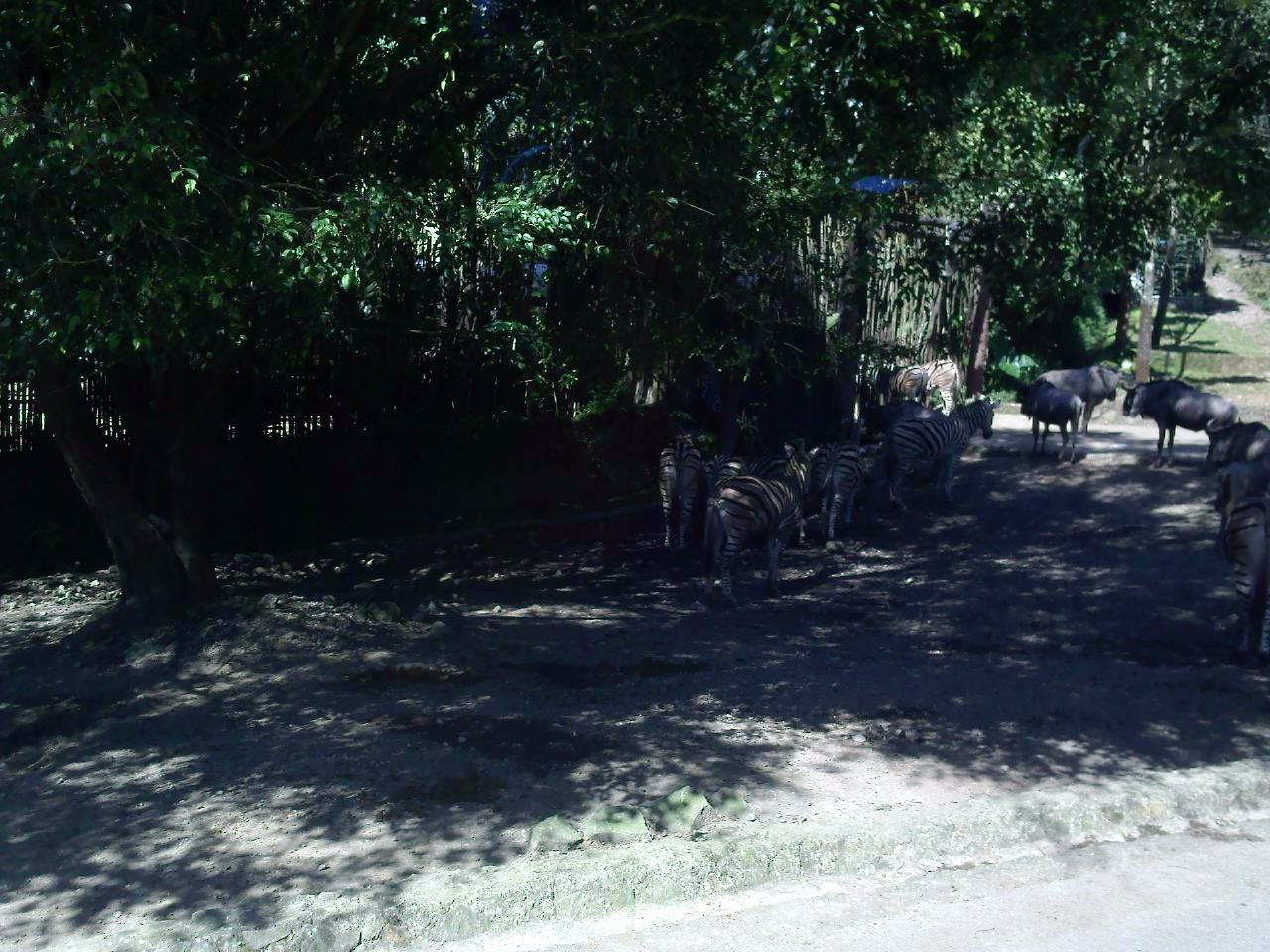This photograph, capturing a scene from a possible zoo or safari park, shows an area viewed from an elevated angle. At the forefront, there is a sunlit patch of grayish ground, while the background reveals tall, leafy green trees casting substantial shadows. The shadows dominate most of the area, obscuring some details but not the distinctive black and white stripes of zebras clustered under the shade on the right side of the image. Among the zebras, there are also other animals, likely wildebeest or bison, with horns, adding to the diversity of the scene. These animals are similarly utilizing the shade, underscoring the heat of the day. Behind the trees, hints of a fence barely peek through the dense foliage, suggesting a contained environment like a zoo or safari park, reinforcing the idea with the suggestion of a road or pathway for vehicles. The overall composition points to a tranquil resting zone for the animals, away from visitor areas.